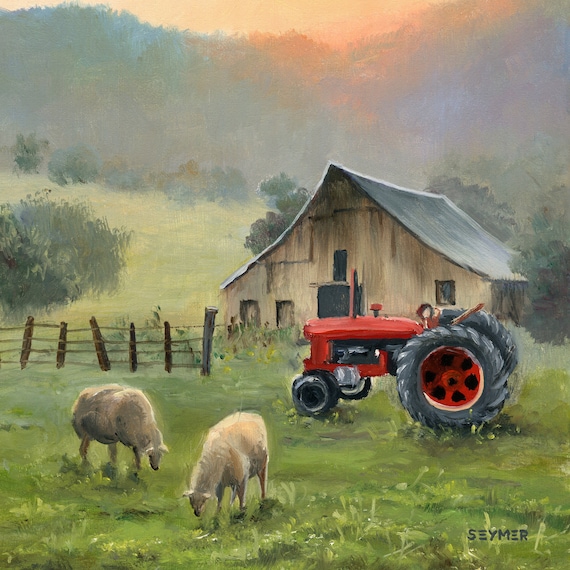The watercolor painting depicts a rural scene with a central barn featuring light brown walls and a dark gray, angled roof. In front of the barn, a small wooden fence encloses a lush field of green grass, extending both behind and in front of the structure. Two light beige sheep are seen grazing with their heads bent down towards the grass, seemingly intent on their meal. Nearby, a tall red tractor with large black wheels at the back and smaller black wheels at the front stands out prominently. The scene is complemented by several dark green bushes or trees in the background, and the sky above is a mix of dark gray hues with a dark orange glow near the top. Additionally, the painting includes a few details such as three windows and a black door on the barn, and the artist's signature, "S E Y M E R," in gray on the bottom right. Overall, the painting captures a tranquil, pastoral atmosphere with attention to detail in both the natural and man-made elements.